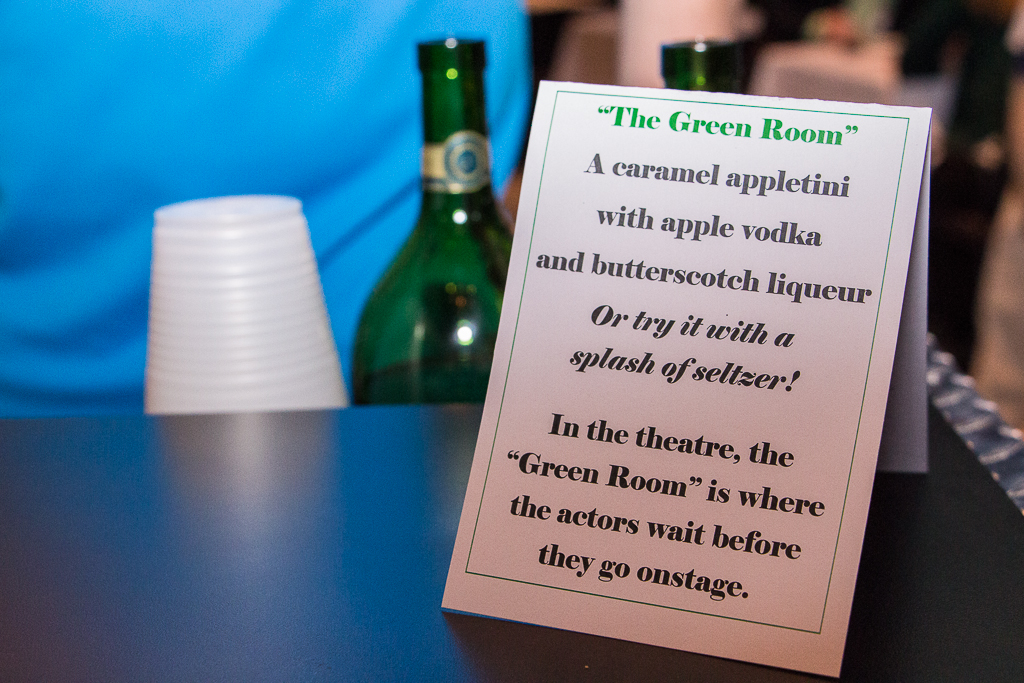The photograph captures a detailed scene featuring a piece of paper standing upright on a black table. The paper serves as a sign and reads "The Green Room" in green text, followed by a description in black text: "A green caramel Appletini with apple vodka and butterscotch liqueur. Or try it with a splash of seltzer." Below this, the sign explains, "In the theater, the green room is where the actors wait before they go on stage." 

Behind the table, the setting reveals several objects, including an upside-down plastic cup and a couple of green bottles likely containing wine or liquor. These items are set against a blurry background where a person in a blue shirt can be seen standing. Additionally, on the right side of the table, there may be some cans, potentially seltzer, although they are somewhat unclear and blurry.

The scene includes a variety of colors such as light blue, white, green, gold, brown, and pink, and gives an impression of being well-organized. The overall setting appears to be indoors, potentially in a bar, and is bright and clear due to natural light.